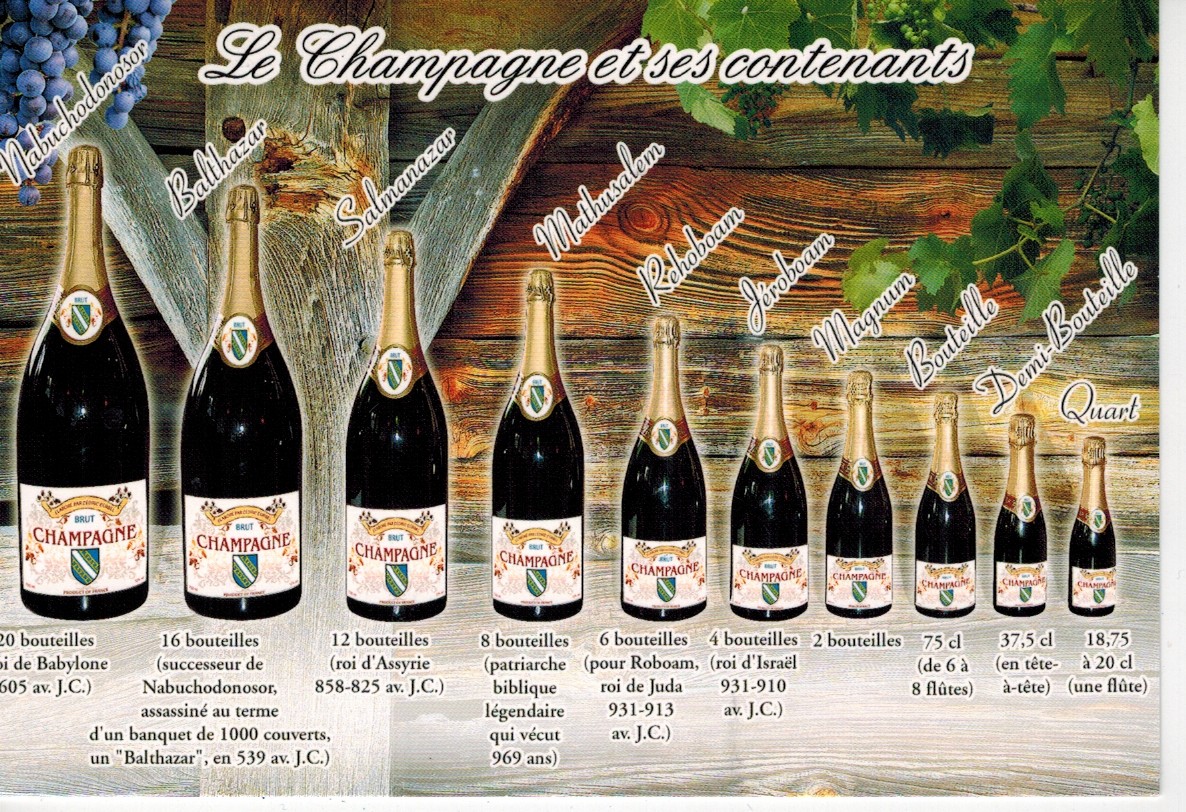This color advertisement for champagne features a rustic wooden backdrop, characterized by grainy barn wood in shades of gray and red, weathered in some areas. The top corners of the image are framed with grapevine leaves, with two bunches of blue or purple grapes hanging down from the top left corner. The title "Le Champagne Essai Contenance" is prominently displayed at the top in French.

Below the title, ten champagne bottles are arranged horizontally, descending in size from left to right. The largest bottle on the left is labeled "Nebuchodonosor," while subsequent bottles are named accordingly: Balthazar, Salmanazar, Mathusalem, Rehoboam, Jeroboam, Magnum, Bouteille, Demi Bouteille, and Quart. Each bottle features a whitish label with the word "Brut" (denoting a dry champagne) over a yellow ribbon, and a green shield with a white sash underneath the word "Champagne." These bottles also have a similar seal at the base of the neck, covered in gold foil.

The ad provides detailed volume measurements beneath each bottle in French. Starting with the largest bottle at 20 Bouteilles down to the smallest at 18.75 CL, these quantities are presumably in liters, milliliters, or another unit of volume. Additional descriptions indicate that the smallest bottle can fill 8 flutes of champagne. The names of the bottles are written in black cursive, diagonally from the lower left to the upper right above each corresponding bottle.